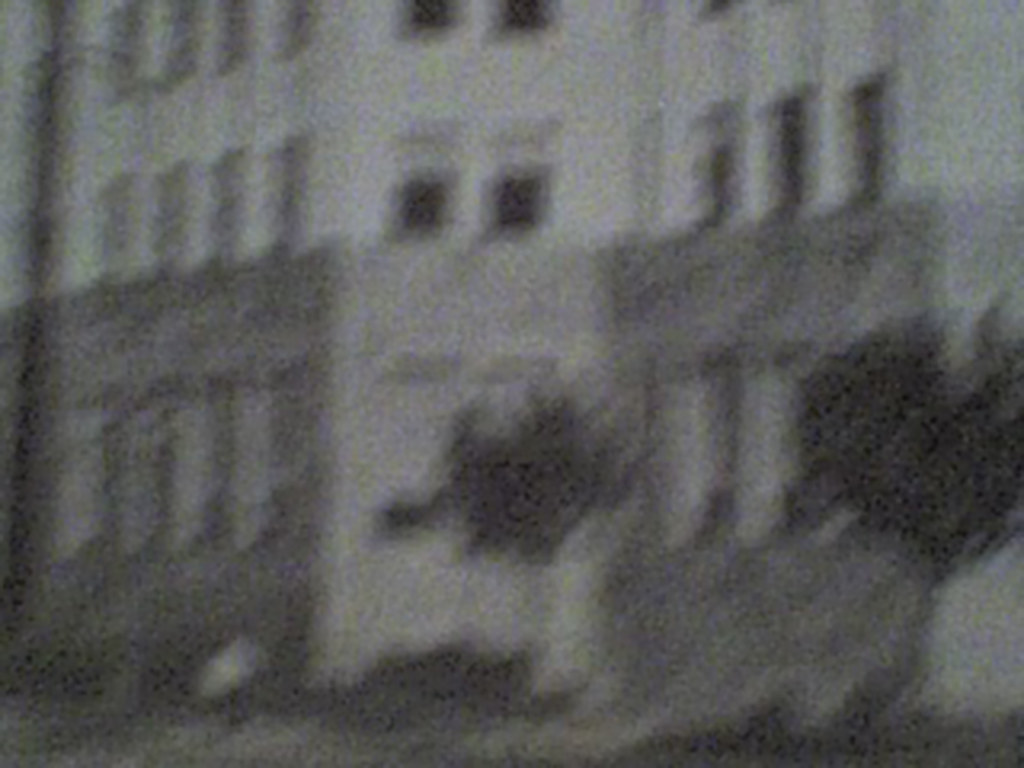A grainy, low-resolution black and white photograph depicts an old, white building. The image appears to be from a bygone era, characterized by its blurry, vintage quality. At the bottom of the building, a central grayish segment is flanked by darker gray areas on both the left and right sides. Above this section, the façade is adorned with numerous windows, more distinctly visible in the middle. The windows here seem to be facing directly towards the viewer. On the bottom right, indistinct black shapes resembling bushes or trees are present. Additionally, a pole is visible to the left side of the image, adding to the historical ambiance of the scene.